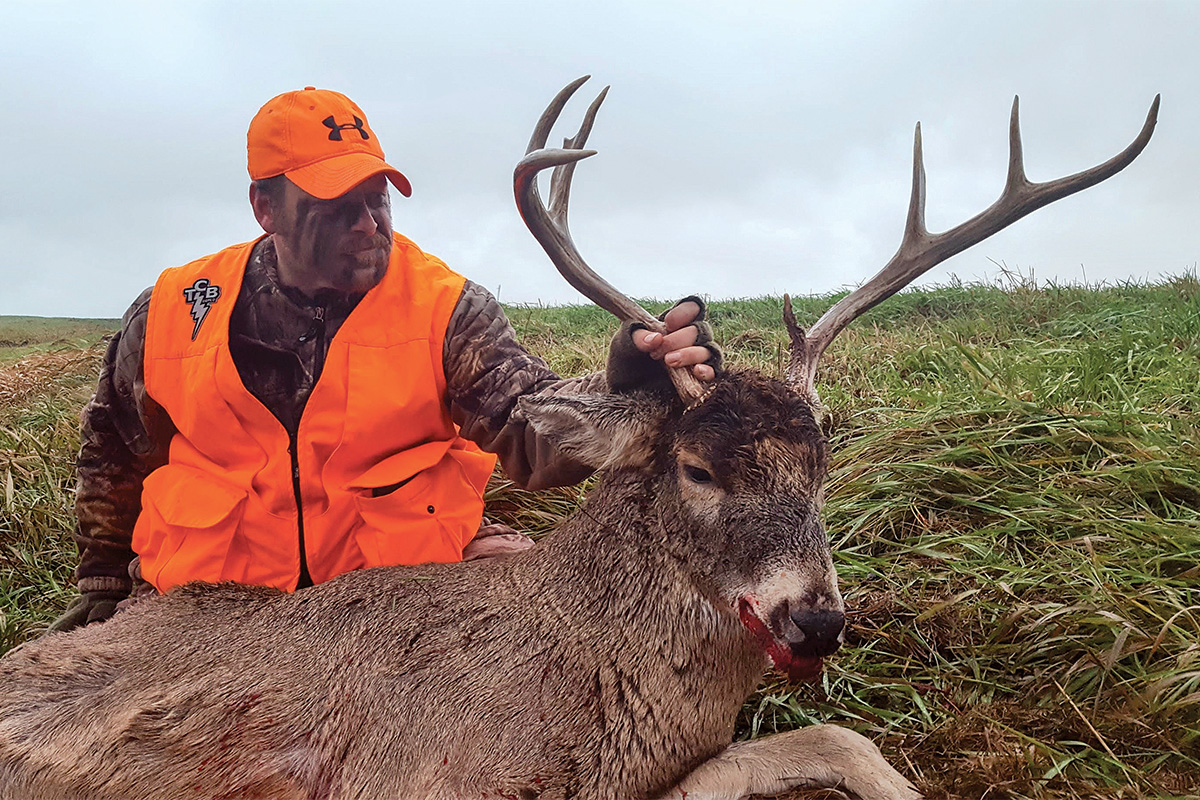In the photograph, a hunter is prominently featured in a daytime outdoor setting under a gray, gloomy sky. The man is dressed in a camouflage jacket with face paint, a bright orange cap with an "H" on it, and a yellow vest adorned with several pockets and marked with "TCB" and a lightning bolt. He is crouched behind a dead buck (deer) with brown fur, which is laying on the ground in front of him. The hunter firmly grips one of the deer’s antlers with his left hand, positioning the animal’s head to face the camera. The deer’s eyes are open, and there is visible blood pouring from its mouth. The background features a green grass field, emphasizing the natural setting of the hunt. The clear and well-lit image captures the detailed attire of the hunter and the somberness of the scene.